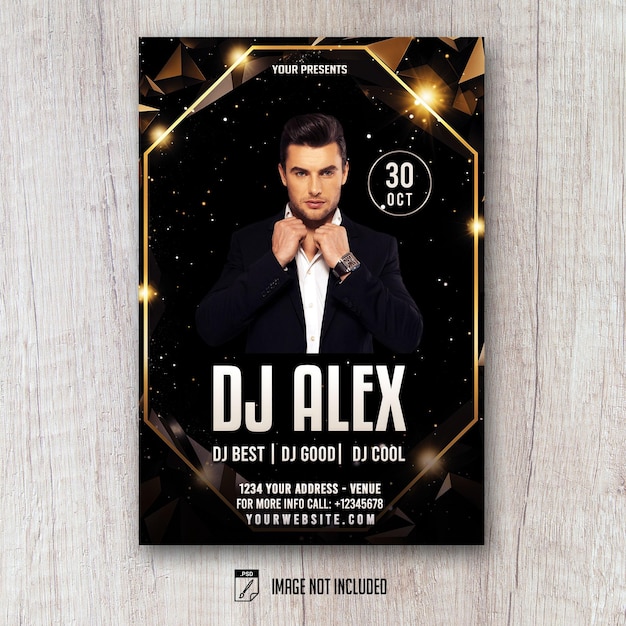The poster advertises a show featuring DJ Alex. It is rectangular, approximately 3 inches high and 2 inches wide, displayed against a light-toned wooden wall with either vertical or horizontal slats having a whitish hue and a slight reddish-pink undertone. The poster itself is predominantly black, adorned with small star-like lights on the background. At the top, in white print, it reads "YOUR PRESENTS." Below this title, there is a striking image of a young man, around 23-24 years old, with light brown skin and slicked-back black hair. He is dressed in a black suit jacket over a white collared shirt, without a tie, and is adjusting his collar, showing off his watch. He appears slightly unshaven. Surrounding him, a gold hexagon outlines his figure, adding a geometric appeal. The corners of the poster feature gold geometric shapes, resembling triangles or pyramids. Over his left shoulder, the date "30 OCT" is printed. Below his image, the text states, "DJ Alex" followed by "DJ Best, DJ Good, DJ Cool" arranged side by side. At the bottom, contact details are provided: "1234 Your Address, Your Venue. For more info call +12345678. Yourwebsite.com." Additionally, "image not included" is noted outside the poster's border on the wooden background.